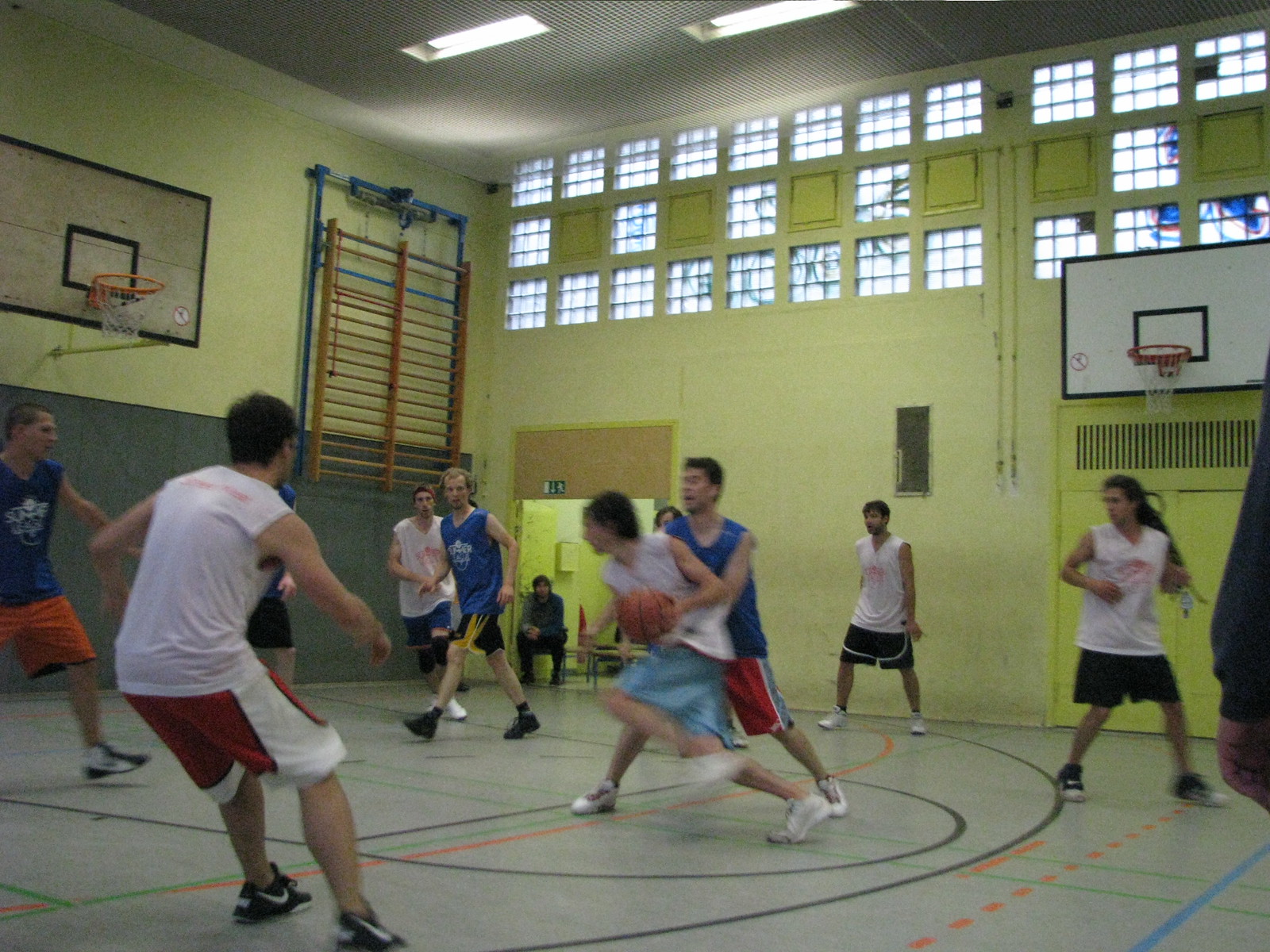The image depicts an indoor gymnasium with yellow walls adorned with multiple square windows arranged in three rows, some of which are partially blocked with yellow panels. The gym's tan basketball court features black, green, and orange lines. Several young men, appearing to be in their early 20s, play basketball in street clothes, not team uniforms, with a variety of sleeveless shirts and knee-length shorts in different colors such as blue, white, red, and black. At the center of the action, a player in a white shirt and blue shorts is driving towards the basket with the ball, pursued by another player in a blue shirt and red shorts. Both appear slightly blurred due to motion. Two basketball hoops, one on each wall visible in the image, have white backboards featuring black squares and standard rims and nets. Additionally, on the left wall, beside one of the hoops, are metal rungs resembling ladders, colored orange. In the corner on the sideline, a man in a gray shirt and black pants with dark hair sits on a chair, observing the game.